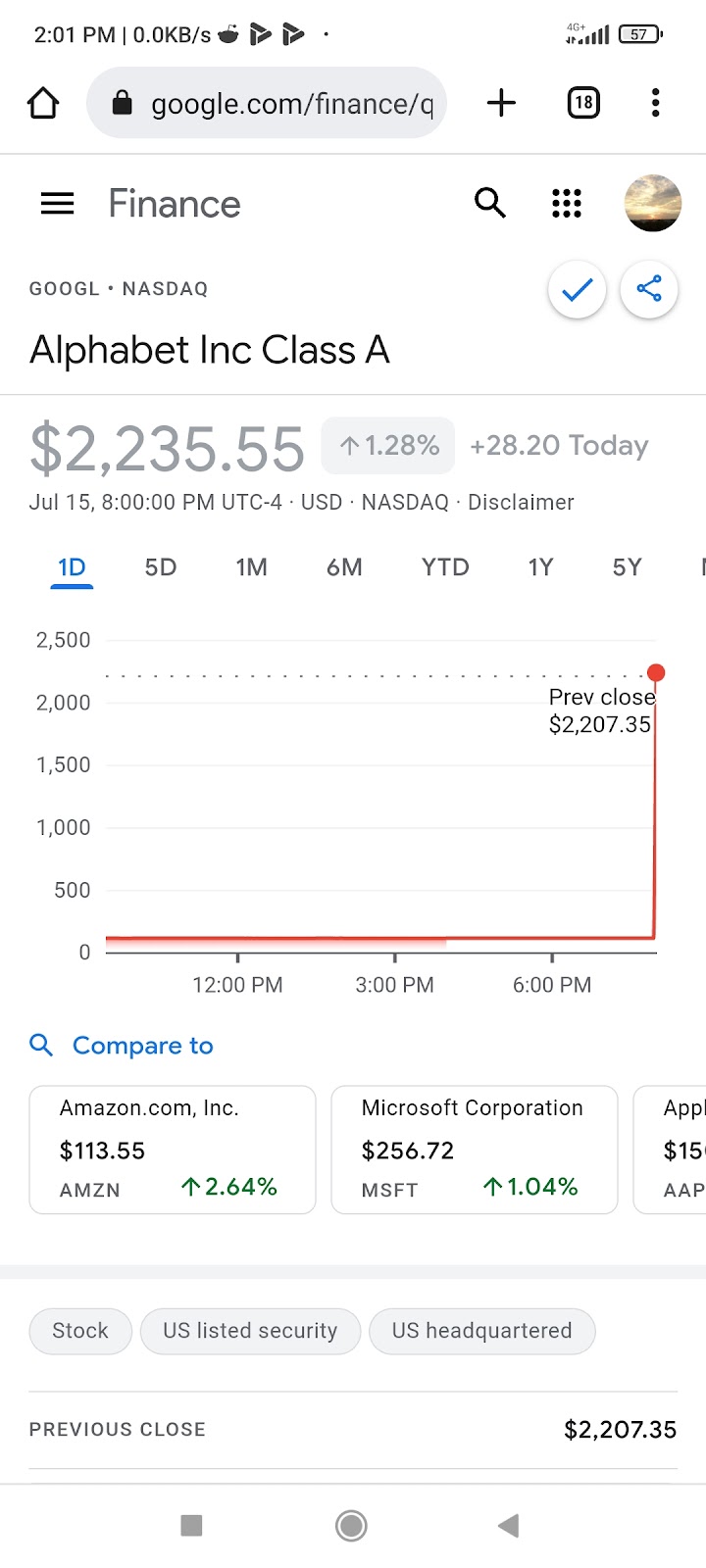The image is a screenshot from a cell phone displaying a Google search results page focused on financial data. The background is primarily white with varying text colors including black, gray, blue, and green. 

In the top-left corner, the time reads 2:01 p.m. Accompanying this are additional icons and text indicating 0.0 kilobytes per second, the Reddit logo, and two triangular-shaped logos. 

On the top-right corner, icons for 4G connectivity, reception bars, and a battery status at 57% are visible. The URL in the search bar at the top is truncated but reveals the beginning string "google.com/finance/Q."

The page indicates that there are 18 other tabs open on this device. The content of the page focuses on financial information with the word "Finance" prominently displayed. Beneath it, "Google Nasdaq" and "Alphabet Inc. Class A" are noted, along with the stock price of $2,235.55.

A line graph is presented below this information, charting the stock value (y-axis) over time (x-axis) with specific markers labeled for 12 p.m., 3 p.m., and 6 p.m.